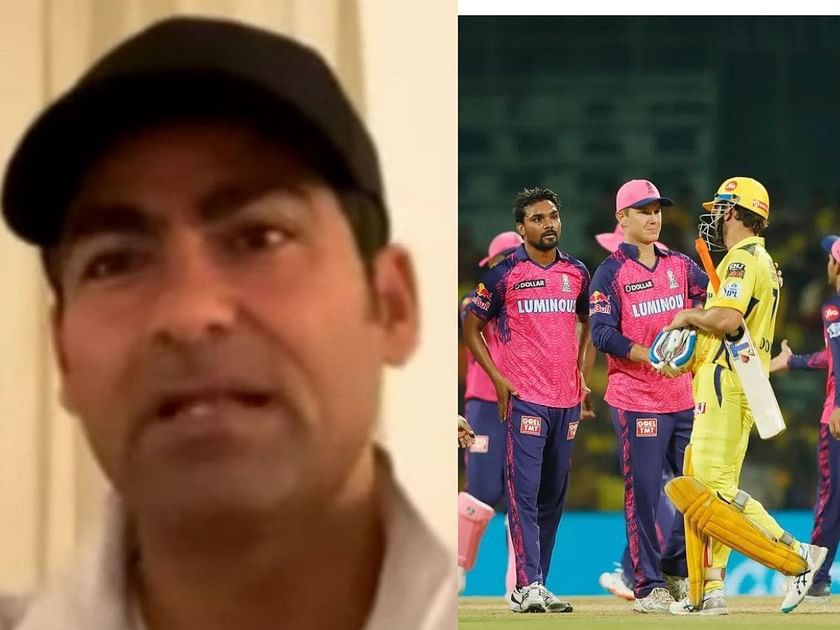This composite image features two distinct photographs arranged side by side. The left side showcases a close-up headshot of a man with Spanish features: dark skin, prominent dark eyebrows, and deep-set dark eyes. He is wearing a black hat and a white collared shirt. His mouth is open, revealing his teeth, capturing a moment of expression.

On the right side, we observe a scene from what appears to be a sports game, specifically cricket based on the equipment and attire. In the foreground, a man dressed in a yellow jersey and helmet is holding a cricket bat. He is shaking hands with a player from the opposing team, who is wearing a pink and purple jersey and a pink hat. Surrounding them are other players from the same team, all clad in matching pink and purple uniforms, indicating a moment of camaraderie or sportsmanship on the field.